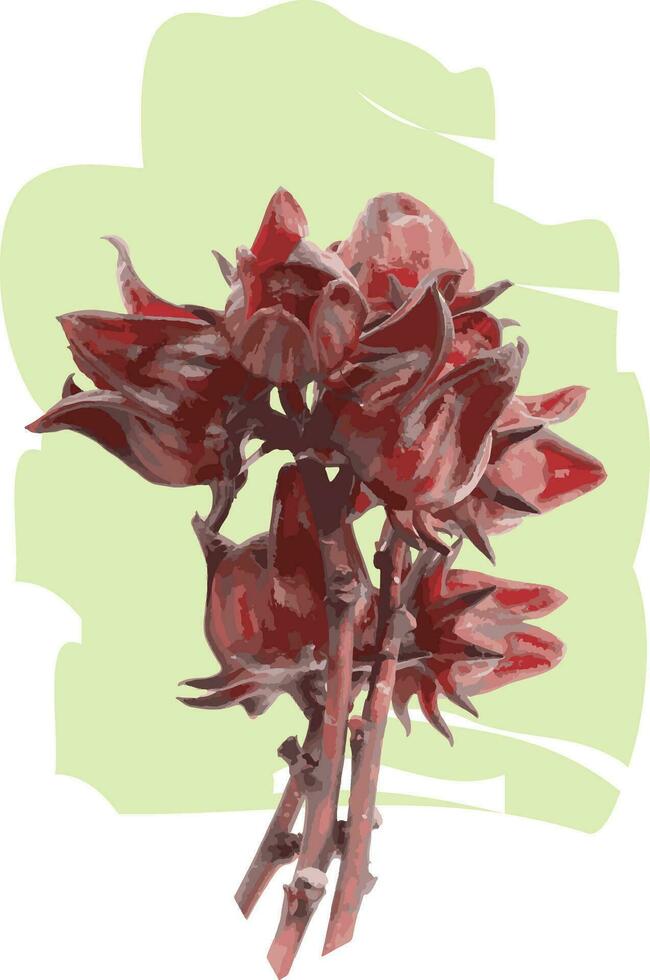This digital rendering presents a painting of red flowers set against a green and white, splotched background. The background features an abstract shape with light green tones interspersed with white. In the foreground, three thick, woody stems emerge, each supporting multiple red flowers. There are approximately eight flowers in total, each boasting five petals that are not fully open, resembling a cross between tulips and roses. Interestingly, the stems are also red rather than the typical green. The overall composition gives an impression of digitally-rendered artwork with an eye-catching, if somewhat messy, background that might be found displayed in an art gallery.